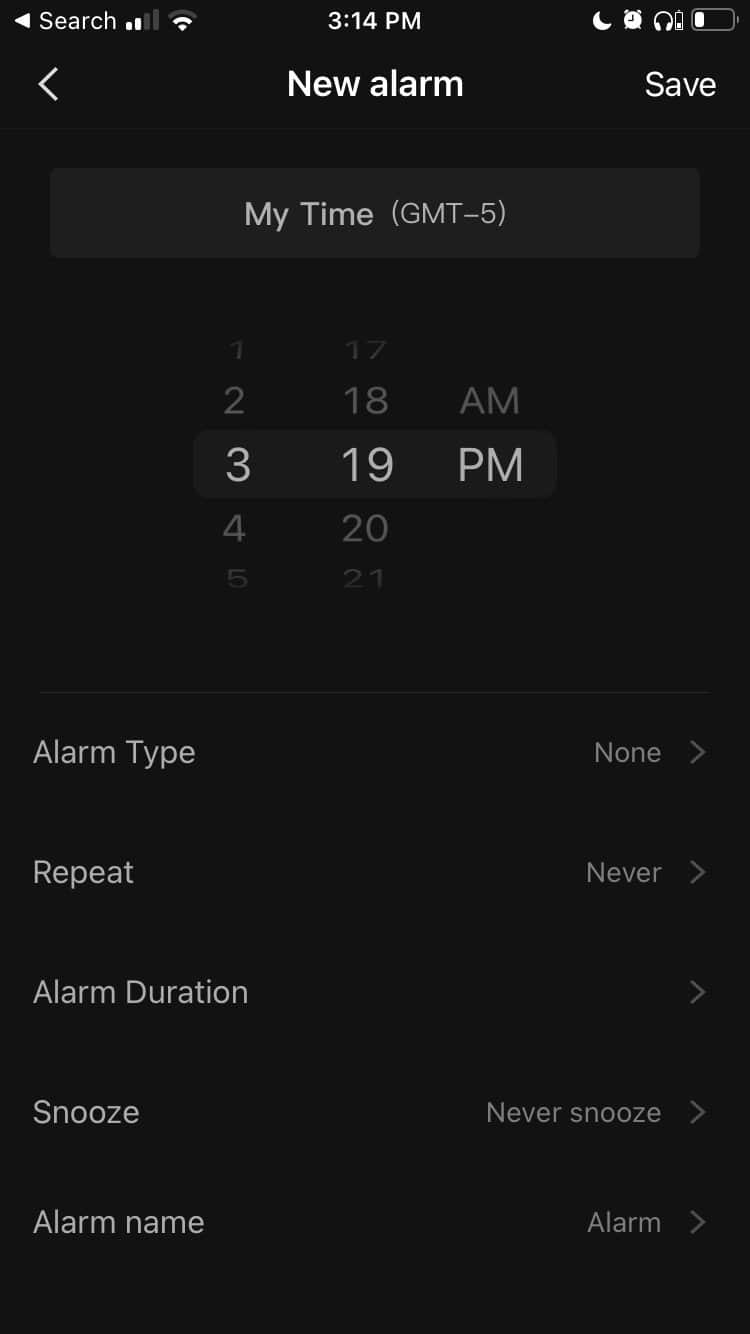A detailed photo of a smartphone screenshot showcasing the interface to set a new alarm. The image is in portrait orientation with a black background, and is approximately twice as tall as it is wide, matching typical smartphone screen proportions. At the very top is a black status bar featuring various white icons and text: a left-pointing arrow, the word "Search," followed by a signal strength icon showing two out of four bars, a Wi-Fi icon missing its top bar, the current time displayed as 3:14 PM, and icons for ‘Do Not Disturb’ (moon), an alarm clock, headphones, and a battery icon indicating a low charge level. Below this, there is a lighter gray header with a left-back caret, followed by the text “New Alarm” and a “Save” button in a thinner, white font. 

The main section of the screenshot has a middle gray box containing the text “My Time GMT-5.” Below it, there is an interactive wheel-like scrolling interface to set the hours and minutes for the alarm. The hours are numbered from 1 to 5 on the left, with selectable minutes from 17 to 21, and a designation for AM or PM, with PM currently highlighted and the time set to 3:19 PM. Beneath this scrolling interface, various alarm settings options are listed, including "Alarm Type," "Repeat," "Alarm Duration," "Snooze," and "Alarm Time," indicating the adjustable parameters for the alarm.